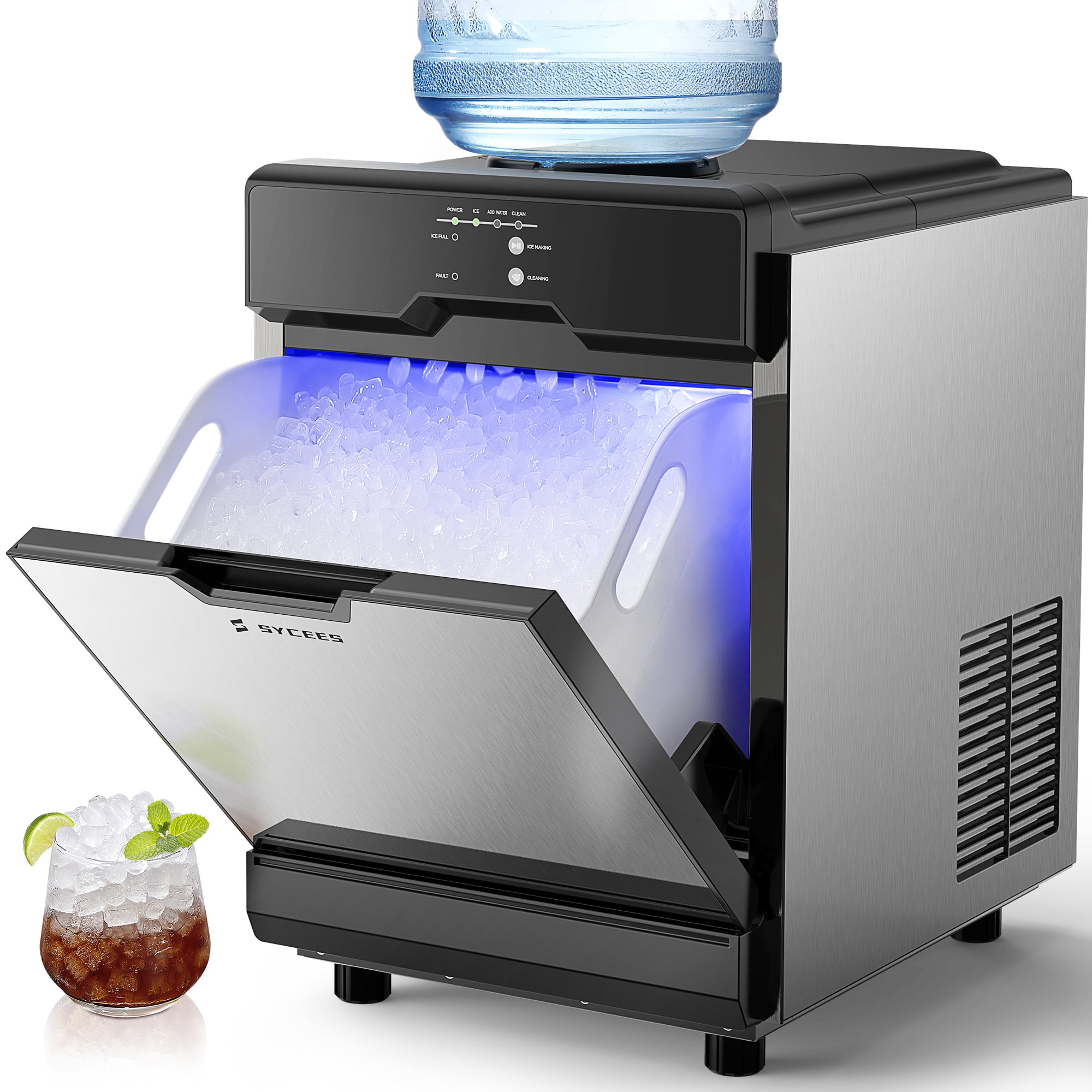This photograph captures an advanced ice maker with a built-in water dispenser, situated in front of a striking ultraviolet blue background. The ice maker, designed as a sleek silver metal cube, features black plastic fittings and sturdy legs. The front door of the ice maker is open, revealing a drawer brimming with ice cubes, some of which are being dispensed in an action shot. At the top of the unit rests a control panel with gray push buttons, and positioned above it is a large, clear Culligan-style multi-gallon water bottle that gives a subtle blue hue.

In the foreground, a large clear glass filled with ice is placed beside the unit on the floor. The glass contains a cola-like beverage occupying the bottom half, while a vibrant slice of lime peers from the left edge of the rim and a fresh sprig of green mint adds a pop of color on the right. The detailed elements and contrasting hues create a visually appealing and refreshing scene.